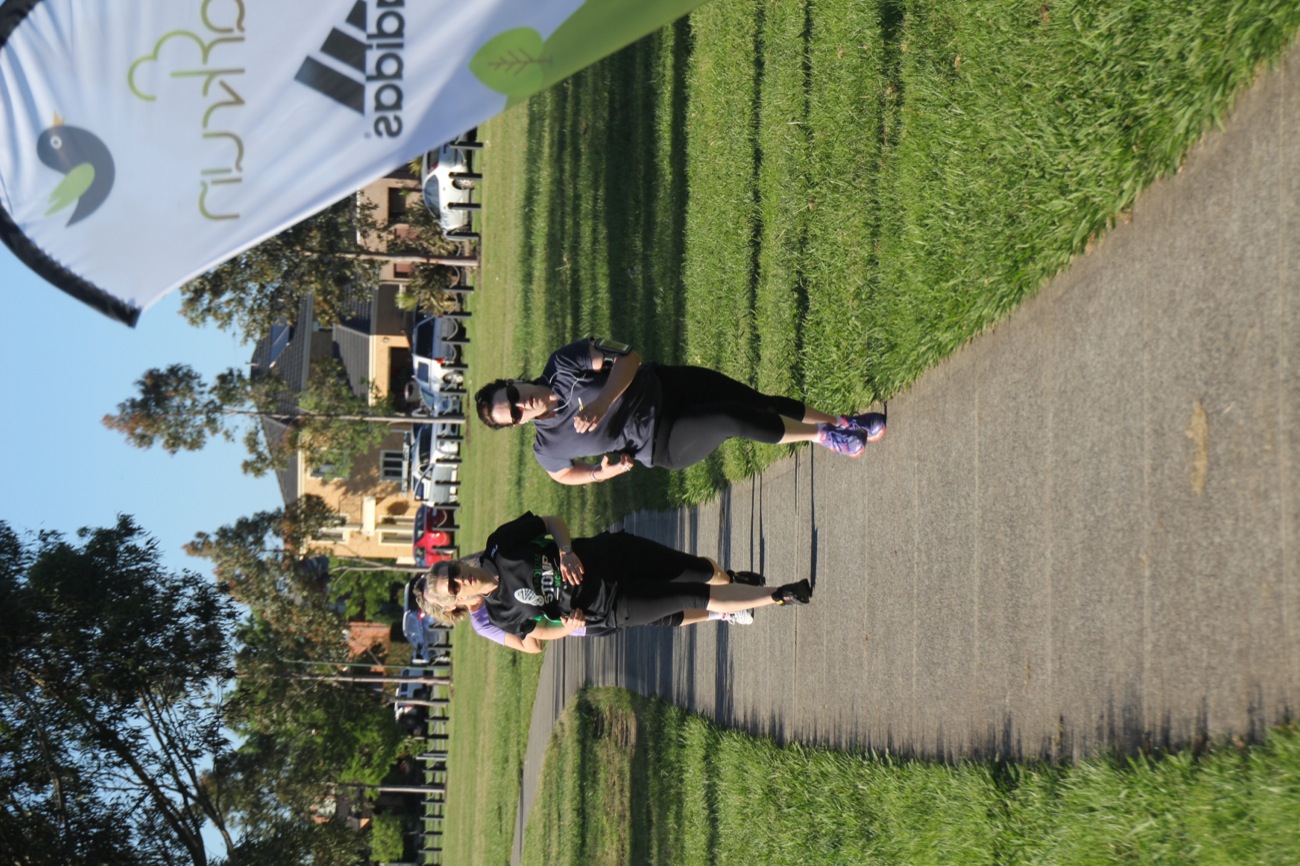This detailed photograph captures the vibrant atmosphere of a park on a sunny day, featuring three women running along a narrow, paved concrete path bordered by green grass. The central focus is on the runners, vividly portrayed in their athletic gear. The woman in the foreground, with dark hair pulled back and sunglasses, wears a gray shirt and black knee-length leggings; her running posture is dynamic, left arm forward with a semi-clenched fist and the right arm back with an open hand. Behind her, a blonde-haired woman with sunglasses and a black outfit follows, also in a vigorous stride with her left arm bent forward. A third runner is partly obscured behind the second woman, identifiable by her presence but not her distinguishing features. 

In the background, the park scene extends with lush trees predominantly on the upper left, creating a serene natural environment. Additionally, a brick building and parked cars are visible, suggesting a busy yet peaceful urban park. A partly-visible banner with the Adidas logo and a picture of a bird on the upper right hints at a possible organized event, though the casual running attire of the women suggests it's not a formal race. The long shadows cast on the ground and the bright blue sky indicate that the photo was likely taken either early in the morning or later in the afternoon, further enriching this picturesque capture of a day at the park.